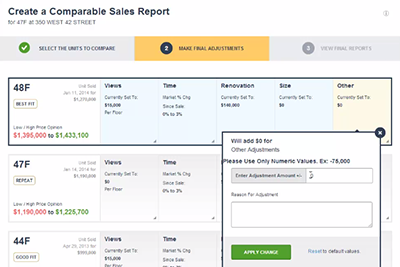The image shows a complex user interface for creating a comparable sales report. On the left side of the interface, there's a label that reads "4173 Fifty West 42nd Street." Below this, there are two tabs: one labeled "Units / Companies" and the other "Adjustments." The image appears to be in poor resolution, making it difficult to read when it's small and not much clearer when enlarged.

Below the tabs, there's a black-bordered rectangle with the text "48 F" on the left side. Inside the rectangle, red text displays the values "$1,395,000" to "$1,433,100" in green, although the purpose of these numbers is unclear. Next to this, there are labels that likely read "Views," "Time," and "Renovations," followed by "Size" and "Owner."

A pop-up appears on the interface with instructions, though it's tough to decipher due to the resolution. It seems to prompt users to "use only numeric values" and to "enter adjustments," but the exact text is not entirely clear.